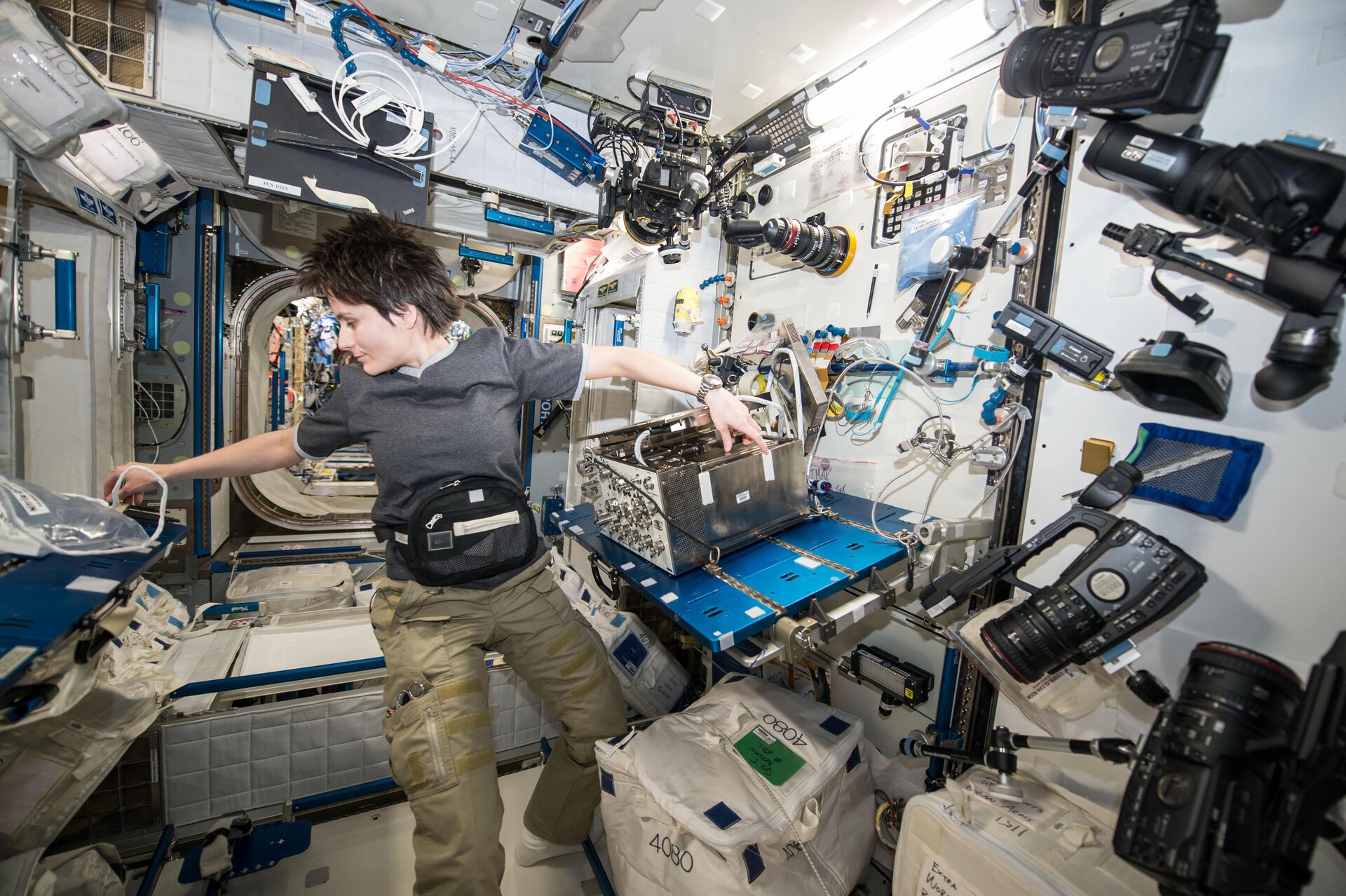In this detailed image of the inside of a compartment in a space capsule, likely the International Space Station, a Caucasian woman with short, spiky, dark brown hair is at the center. She is wearing a gray short-sleeved shirt and tan cargo pants, with a black fanny pack around her waist. On her left wrist, she has a wristwatch. She appears to be leaning towards a wall, reaching for a component or a bag on a shelf, surrounded by a variety of flying cameras and assorted equipment. The compartment features stark white walls and floors, along with blue shelves and handles. A blue shelf supports a silver computer unit that she is working on. The walls are lined with various tools, meters, and black camera equipment. In the lower area of the scene, partially visible, is what seems to be a sofa or bed covered with a beige blanket or comforter. A hatch-like door or airlock is also evident, suggesting access to other parts of the station. The scene is reminiscent of a well-organized, high-tech workshop, emphasizing the intricate and compact environment of space living.